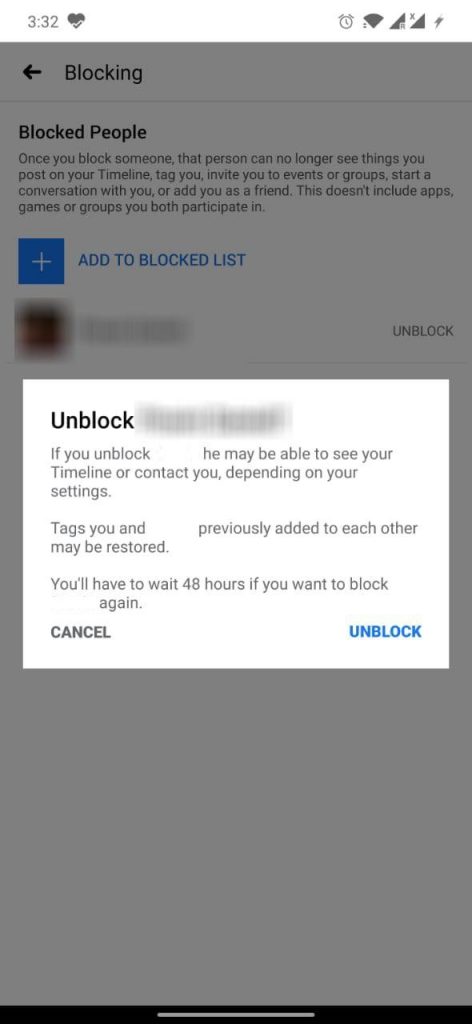This image is a screenshot from a cell phone depicting the options for unblocking someone on Instagram within the app's settings. The top of the screen features a white status bar displaying the current time (3:32) on the left and various symbols on the right indicating an alarm clock, Wi-Fi connectivity, and more.

The main screen itself is greyed out, indicating that a white pop-up dialog box is active in the foreground. At the top of this greyed-out main screen, the title "Blocking" is displayed alongside a back arrow, which allows the user to navigate to the previous page. Below it, the section titled "Blocked People" is visible, with a brief description of its function. There’s also a prominent blue button with a white plus sign labeled "Add to Block List."

Beneath this section, a blurred entry hides the identity of a previously blocked individual. The white pop-up dialog box in the foreground contains the option to unblock this person. Although the name is also blurred for privacy, the text within the dialog provides a cautionary message: "If you unblock [name], they may be able to see your timeline or contact you depending on your settings. Tags you and [name] previously added to each other may be restored. You'll have to wait 48 hours if you want to block [name] again." At the bottom of the pop-up, two selectable options are presented: "Cancel" and "Unblock."

Overall, the screenshot effectively captures the intricate details of the Instagram unblocking interface on a mobile device.